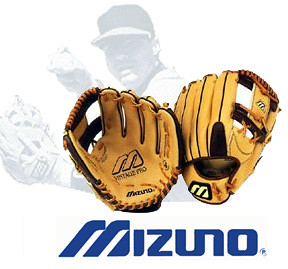This image is a detailed advertisement for Mizuno baseball gloves. Prominently featured are two baseball gloves, displayed in a light tan color with blue borders and brown lacing. One glove shows the palm facing forward while the other shows the palm facing backward, highlighting their design and features. The brand name "Mizuno" is prominently displayed in navy blue at the bottom of the advertisement and also appears on the inside of the gloves. In the background, there is a faintly visible image of a baseball player wearing a cap, holding a baseball aloft in his back hand and preparing to throw with the glove on his front hand. The player adds a dynamic, action-oriented element to the promotional art, making it clear that these gloves are intended for serious play.